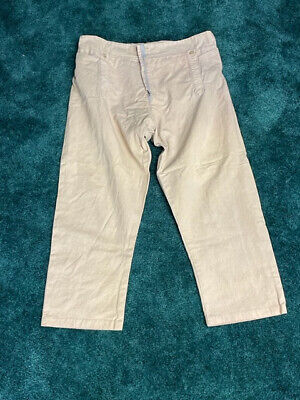This photograph captures a pair of khaki capri pants, laid flat against a contrasting green mottled background. The capris, rendered in a very light tan or off-white shade, feature a defined waistband complete with a fastening button or snap, and a zipper. Notably petite in size, the pants also display metal rivets near the waistband and side pockets. Though the pants are not brand new, exhibiting a slightly weathered appearance and visible fold lines on the legs, they provide a juxtaposition of texture against the deep, dark green of the background.